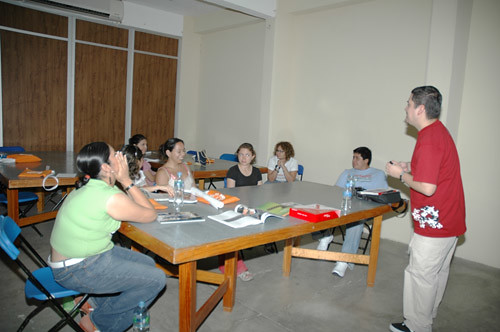The image depicts a lively classroom setting with a man, likely the teacher, standing on the right side of the room. He is wearing a red shirt adorned with holly leaves, khakis, and black shoes, and he has short hair. He engages with a group of seven students who are seated around a large, rectangular table with a gray top and wooden legs, resembling those commonly found in libraries.

Among the students, a girl in a green shirt and blue jeans sits on a blue and black chair, and a boy in a blue shirt with either blue jeans or gray pants and white shoes also participates. There are several others, including one woman who is covering her face with her hands, seemingly laughing, and another who is beaming with a wide smile, both indicating that the man might have just said something amusing. 

The room has beige walls and features wooden elements like doorways or blinds. A secondary table behind the main one also has two girls sitting at it, along with water bottles and open books scattered across both tables. The overall atmosphere is cheerful and engaging, with students visibly amused and attentive to the man standing before them.